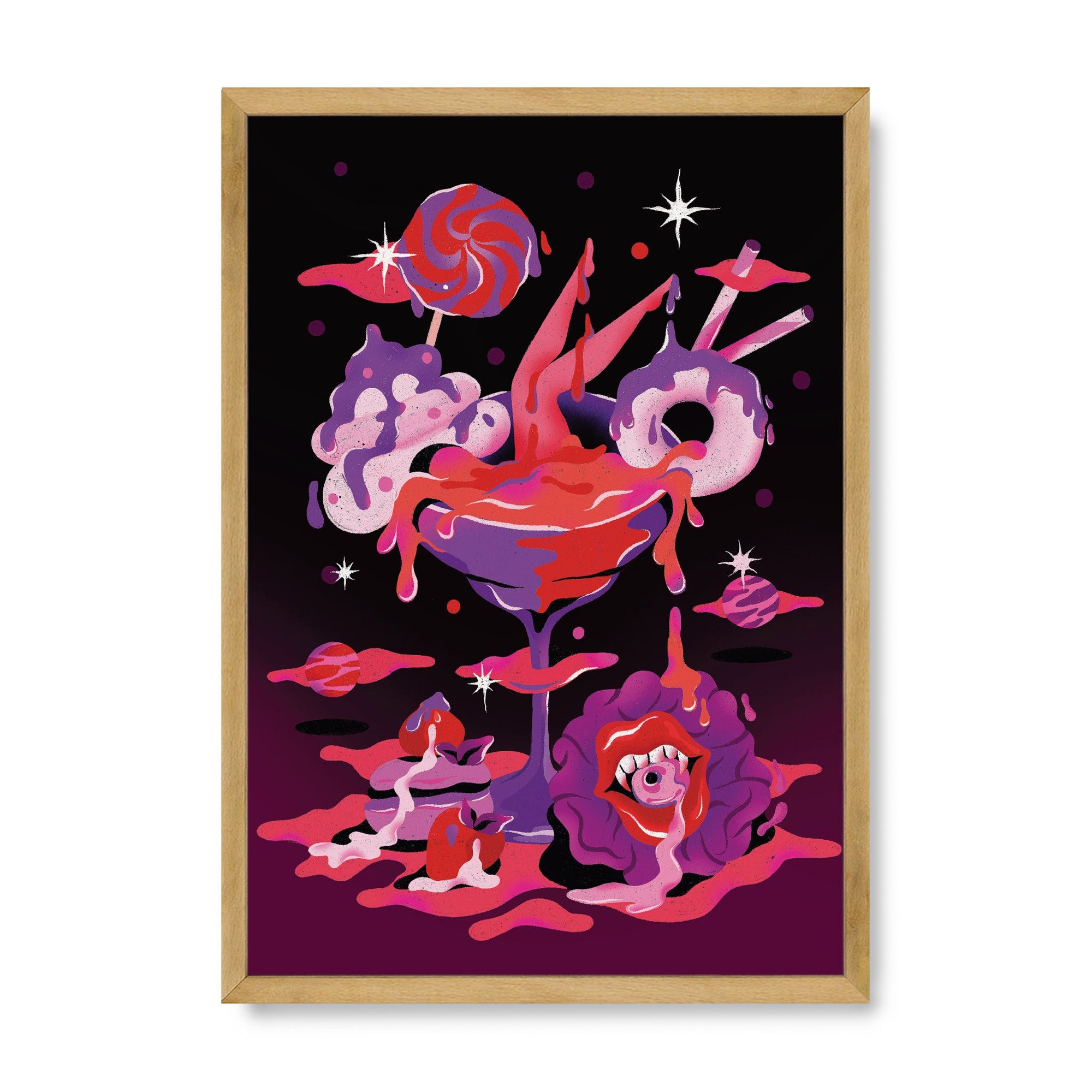The image is a striking piece of abstract artwork resembling a scene from a dream sequence. It is visually trippy and surreal, characterized by a mix of vibrant colors and melting visuals on a predominantly black background that transitions into dark purple hues. The painting is bordered in wood and could be displayed on an 8.5 by 11-inch paper, creating a stark contrast with its black-and-dark-purple canvas.

At the top of the composition, a martini glass is the focal point, filled with rich, red liquid resembling blood, and distinctively, women's legs protrude from it, dripping fluid. Adjacent to the legs is a whipped cream swirl, adding to the bizarre nature of the scene. The glass also contains a melting pink donut covered in purple fluid, accentuating the trippy ambiance. To the right of the glass, there’s another melting donut and an ice cream swirl, implying a sweet yet eerie motif.

Positioned to the bottom of the martini glass is a flower with a mouth that contains vampire-like teeth and an eyeball, enhancing the artwork’s spooky and surreal aesthetic. Scattered around the bottom are additional abstract elements, suggesting fruits like apples embedded in a red, blood-like puddle. A lollipop appears to be melting in the top right, contributing to the cascade of sugary delights draping the scene.

The overall color palette features various shades of pinks, purples, deep maroons, and white, blending seamlessly throughout the drippy and surreal elements. This painting is definitely an artist's creation, devoid of any text, offering a mesmerizing and psychedelic visual experience.